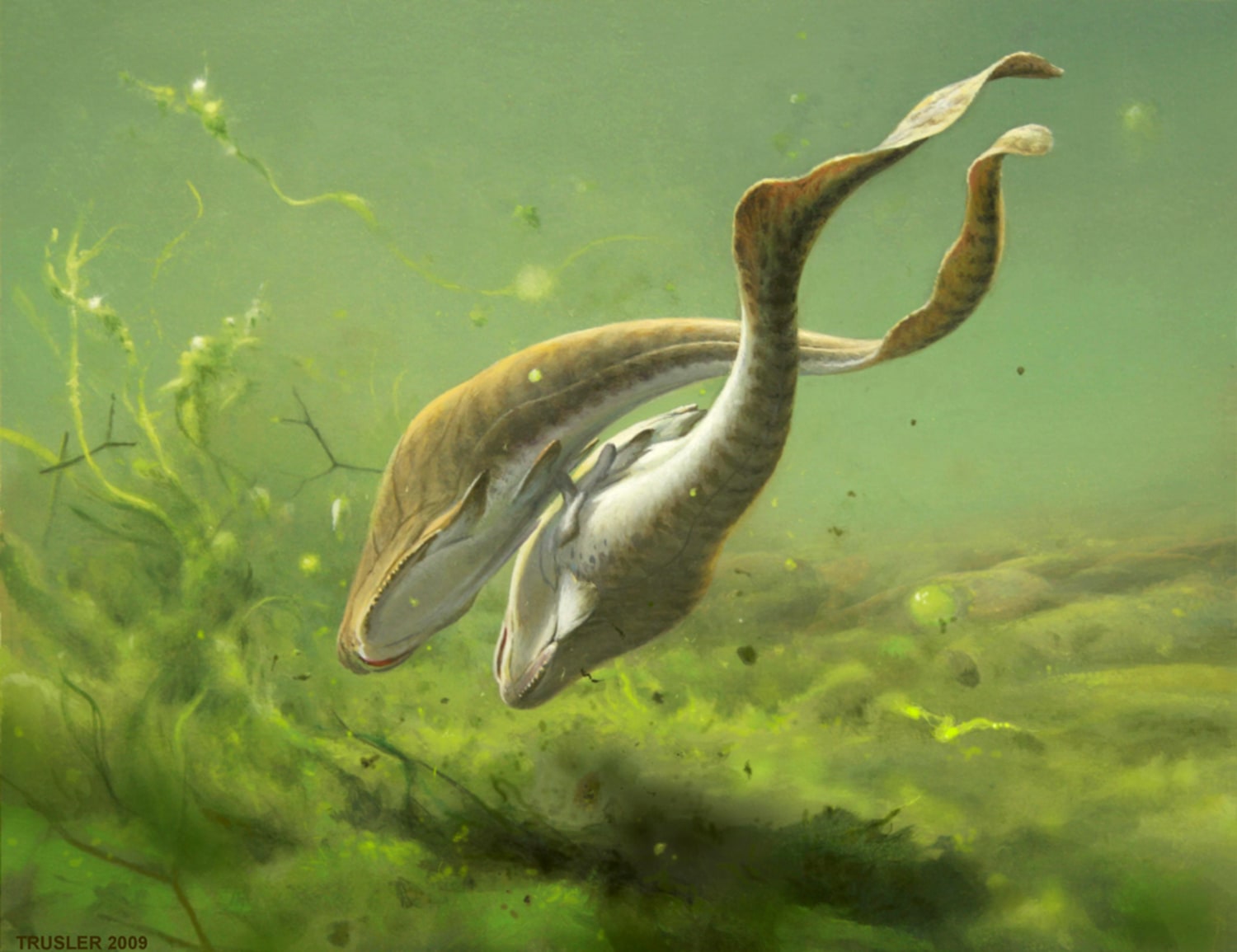The image is a color illustration of an underwater scene in a landscape format, likely a painting or drawing. It features two L-shaped fish, or possibly salamanders, swimming side by side and facing slightly downward toward the murky seabed, which is heavily covered in green algae and plant life. The water is green, suggesting it is rich with algae, and the bottom is densely vegetated, with some of the algae resembling grass that reaches up. Both creatures are brownish with some white, and the image is signed "Trasla 2009" or "Tressler 2009" in the bottom left corner.